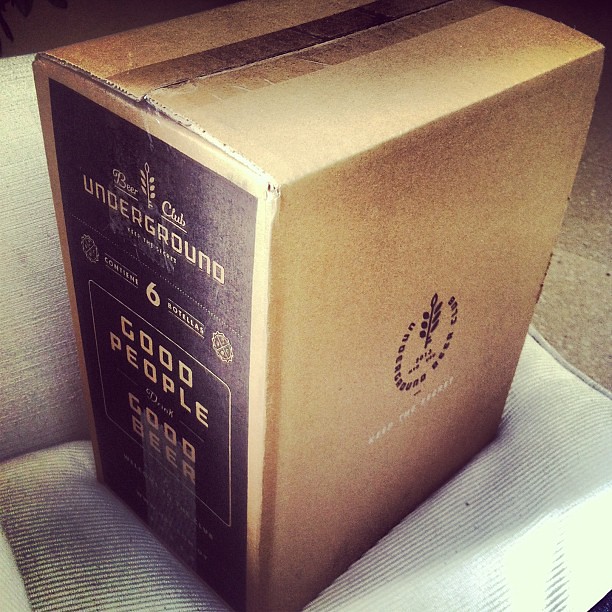In this image, we observe a room with a carpeted floor. Positioned in the center is a sealed, tall cardboard box with tape on both the top and bottom. The box rests on a cushioned piece of furniture, likely a couch with a whitish-gray tint and thin stripes running across it, as well as a backrest. Notably, shadows suggest some light is casting across the scene from an angle.

The box features multiple inscriptions and decorative elements. Prominently displayed on the left side of the box are the words "Beer Club Underground" in capital letters, along with "Good People, Good Beer." Additionally, the phrase "Keep the Secrets" is visible, possibly located towards the bottom of the box. The box design includes a graphic resembling a barley leaf within a circular arrangement of the text. The main colors visible in the room and on the box include shades of white, brown, dark brown, black, silver, and gray. The overall setting appears to be indoors, suggesting the image was taken inside someone's home.